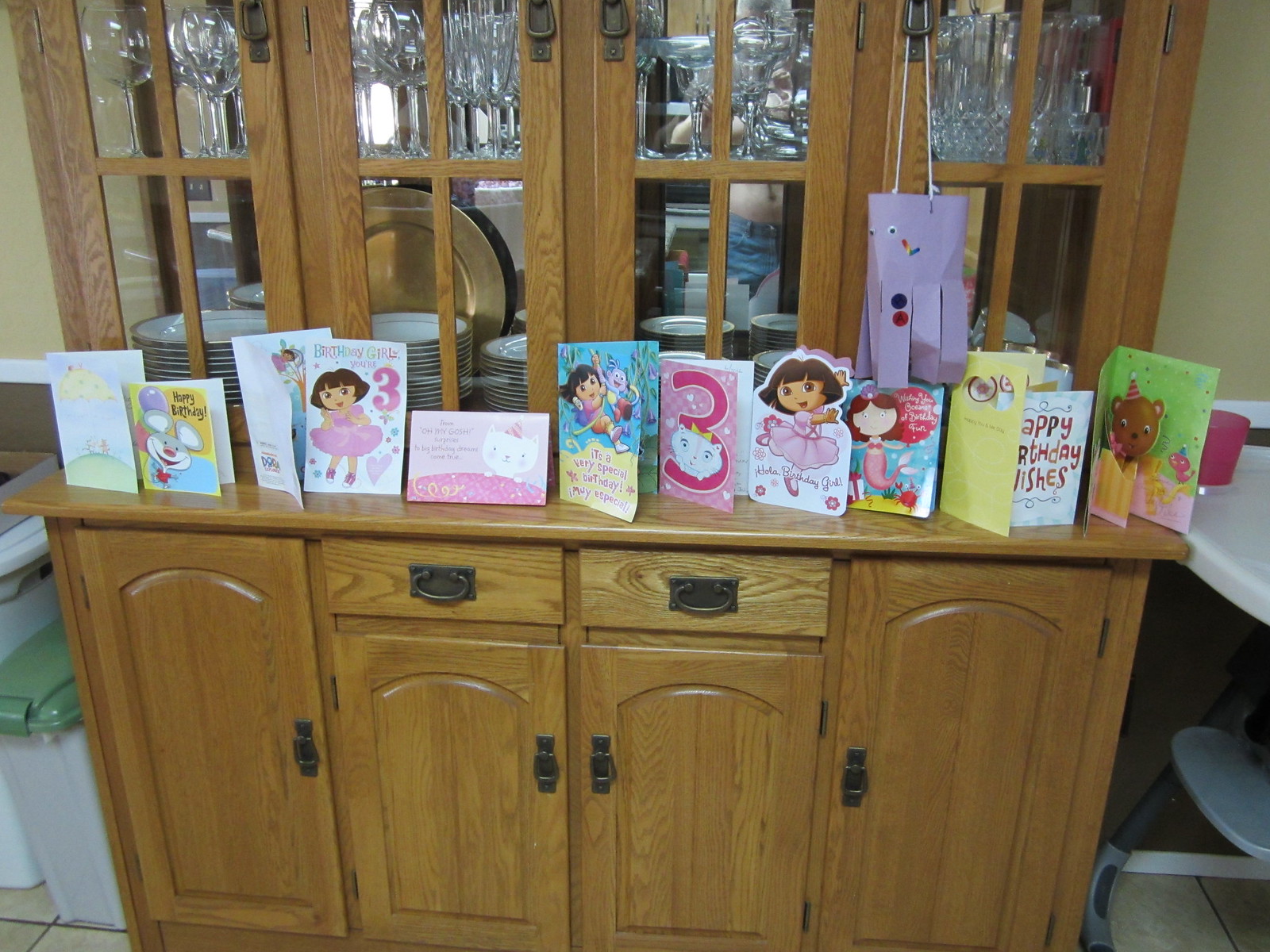This detailed landscape photograph captures a mahogany-hued sideboard in a dining room, richly marked with lighter and darker wood panels. It features a series of storage compartments: two taller cupboards on both ends, two shorter cupboards flanked by drawers in the center, all adorned with dark metal pulls. The top surface of this sideboard is decorated with a collection of birthday cards, arranged in a horizontal display.

The cards predominantly celebrate a little girl's third birthday, as evidenced by multiple cards featuring the number "3". Many cards display anthropomorphized characters of a little girl, often depicted in a pink dress, with some cards bearing the words "Happy Birthday". There's a diversity in design, with various colors and themes including Dora the Explorer, and others with characters and festive illustrations like a rabbit. A standout card is pink and another one on the right side is white, wishing happy birthday, while a yellow one on the left further enhances the festive mood.

Behind these cards, four glass-fronted doors reveal the sideboard's upper section, which contains an assortment of crystal stemware on the top shelf and neatly stacked crockery plates on the bottom shelf. Additionally, a light purple bag with blue and red accents hangs to the left of the sideboard, complementing the overall celebratory atmosphere.